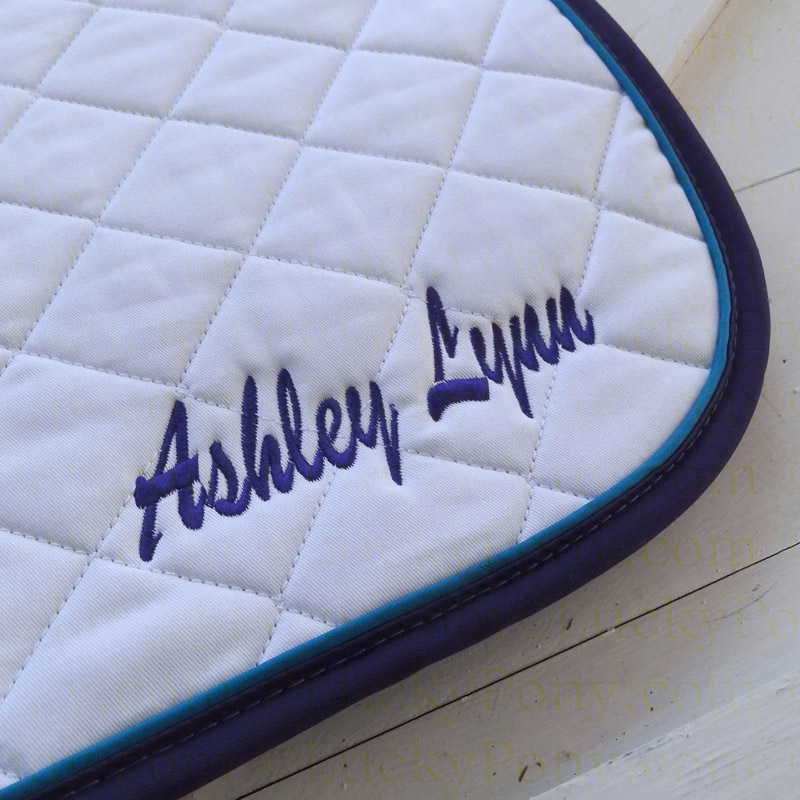The image displays a very close-up view of a quilted fabric piece, set against a white, painted wooden background resembling a table or board. The fabric features intricate white stitching that forms a quilted pattern of squares. The quilted piece is meticulously bound by a dark blue border with a rounded corner and has a lighter blue trim on the inside. In the corner of this quilted fabric, the name "Ashley Lynn" is embroidered in dark blue cursive, with "Ashley" starting with a capital A and "Lynn" starting with a capital L.